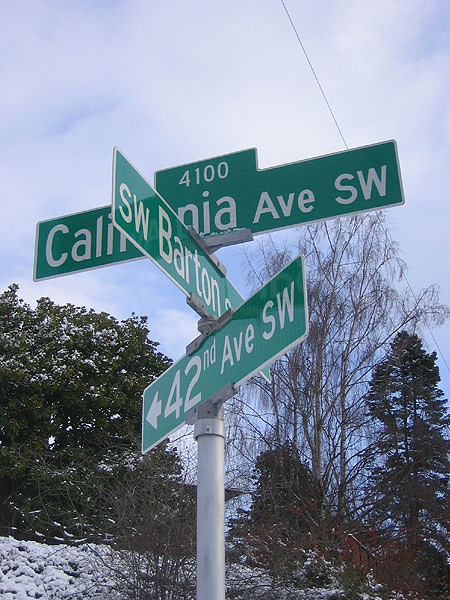This color photograph offers a close-up view of three intersecting street signs mounted on a single gray steel pole. The background showcases a blue, overcast sky framed by leafless trees on both the left and right sides of the image, suggesting a chilly season. Snow lightly covers the ground, just enough for patches of earth to show through the thin layer, hinting at either an early snowfall or a recent thaw.

The focal point is the trio of green, oblong street signs with crisp white lettering. From bottom to top, the signs read: "42nd Avenue SW," "SW Barton Street," and "California Avenue SW," with the top sign also featuring the number "4100" prominently displayed. The clear, organized presentation of the street names and numbers aids in identification and navigation.